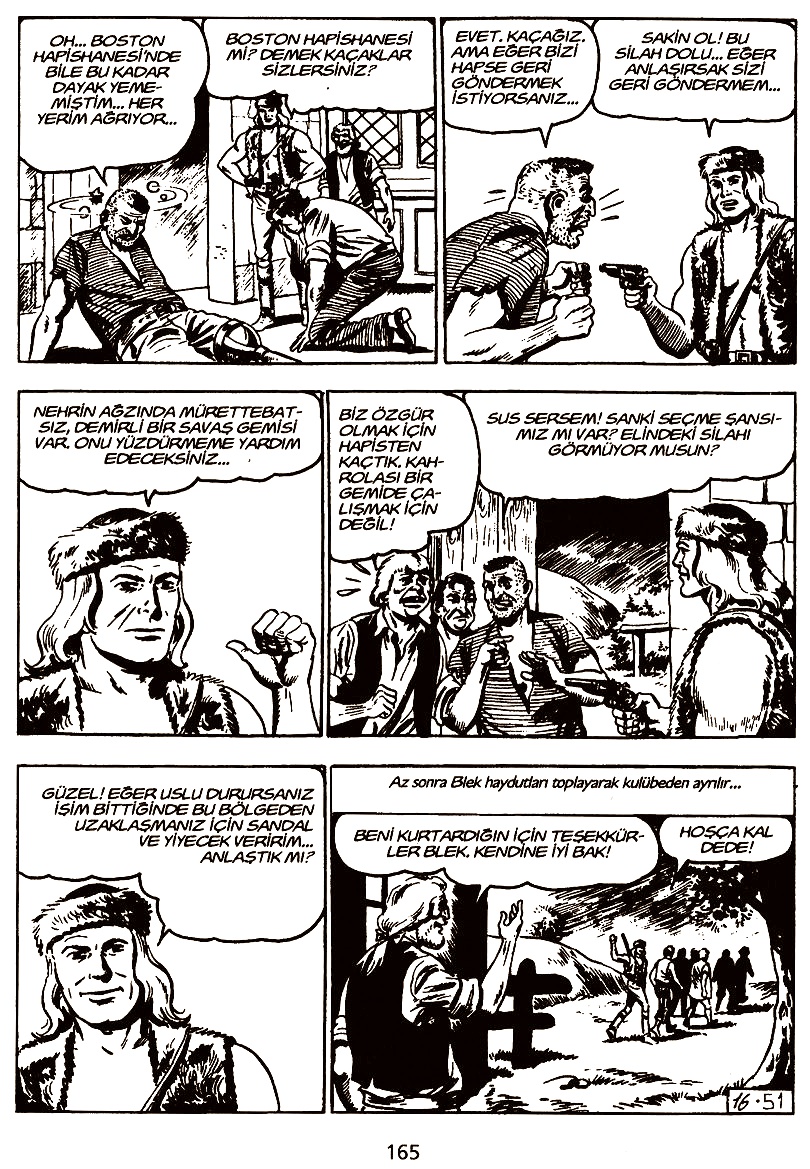This black-and-white comic strip spans six panels and tells a story primarily through the actions of a muscular, shirtless man wearing a fuzzy hat and vest, made to resemble animal hide. The dialogue is in a foreign language, enhancing the comic's mysterious tone. In the first panel, a group of men surrounds another man who is slumped against a wall, dizzy circles spinning around his head, indicating he has been struck or is otherwise incapacitated. The second panel features our main character aiming a gun at another man who appears to be a robber due to his torn, striped shirt. In the third panel on the left, the main character points at himself with his thumb, perhaps asserting his dominance or introducing himself. The fourth panel, on the middle right, displays a conversation between several men, with the protagonist holding his gun up against them, maintaining control. The fifth panel on the bottom left shows the protagonist again, identifiable by his hat and vest, possibly confronting the men. In the final panel, the protagonist waves as a group of men walk away, signaling a resolution of the conflict. Beneath this concluding scene, there is a small, understated number "165," possibly indicating the strip's sequence in a series.